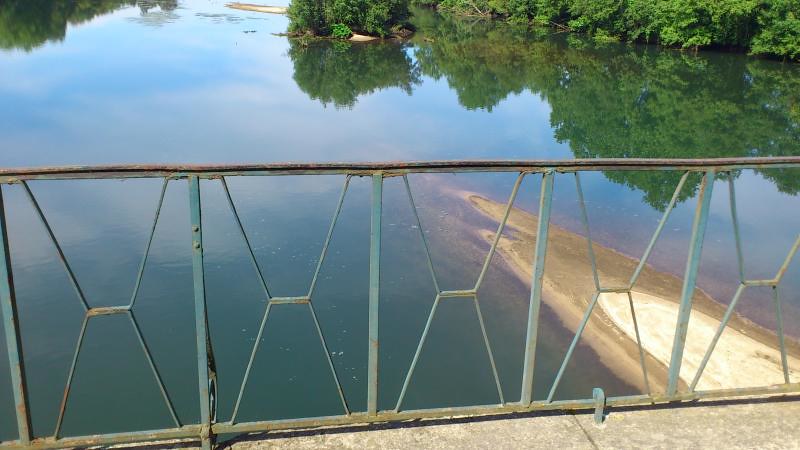This landscape-oriented photograph captures a serene view from a rusted, pale blue metal railing on a bridge, looking out over a tranquil river. The railing, which has sections forming an X shape between the main supports, shows signs of neglect with brown rust adorning its top. Below, the river, a deep turquoise blue tinged with purple and pink hues, winds through the landscape. On the right side, a light brown sandbar juts out into the water, bordered by beige edges. The upper left corner of the image reflects lush green trees, while on the right, a row of trees extends over the river, resembling a mangrove. The tranquil water mirrors the canopy above, suggesting a sunny day. The perspective of the photo, taken from a vantage point high on the bridge, provides a broad view of the land and water below, hinting at the height of the vantage point and the expansive scenery beyond.